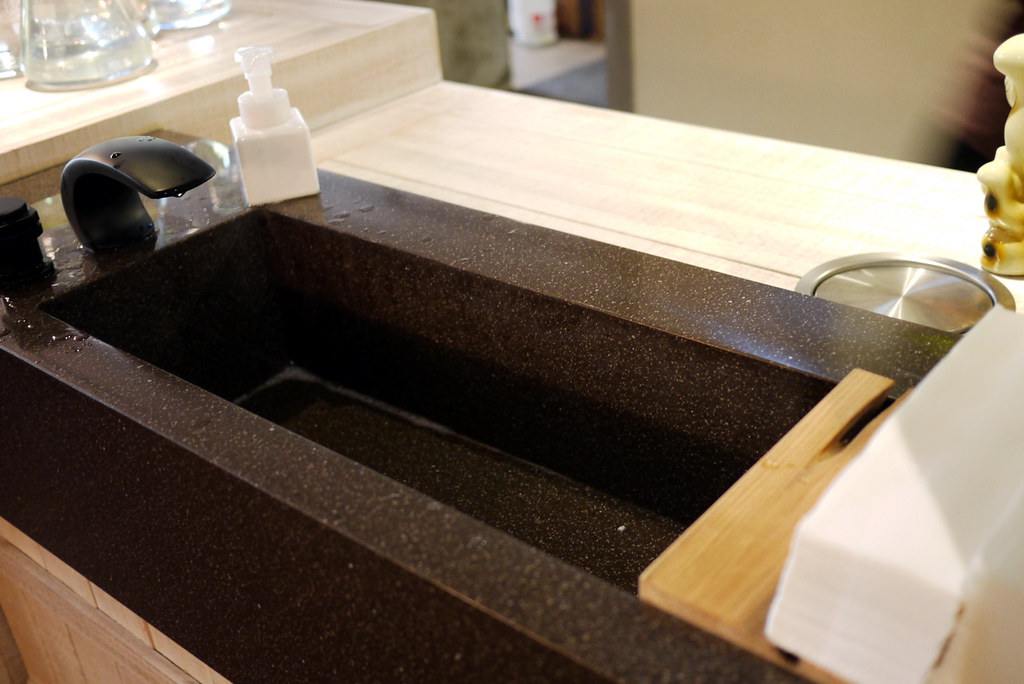This horizontally-oriented color photograph showcases a modern bathroom sink, prominently featured in a diagonal orientation from the top left to the bottom right of the image. The sink, made of an immaculate brown stone or granite, is rectangular and harmoniously nestled in a light-colored wooden shelf. A sleek, black modern faucet with a minimalist curved design is positioned at the upper left corner of the sink, accompanied by a square white soap dispenser. At the bottom right edge of the sink, a wooden board holds a square soap bar, casually placed in alignment with the sink's diagonal orientation. In the background, a slight elevation in the shelf holds several glasses, adding a touch of practicality to the composition. The wall behind features a doorway, through which various blurred objects can be seen, lending a sense of depth and realism to the scene.